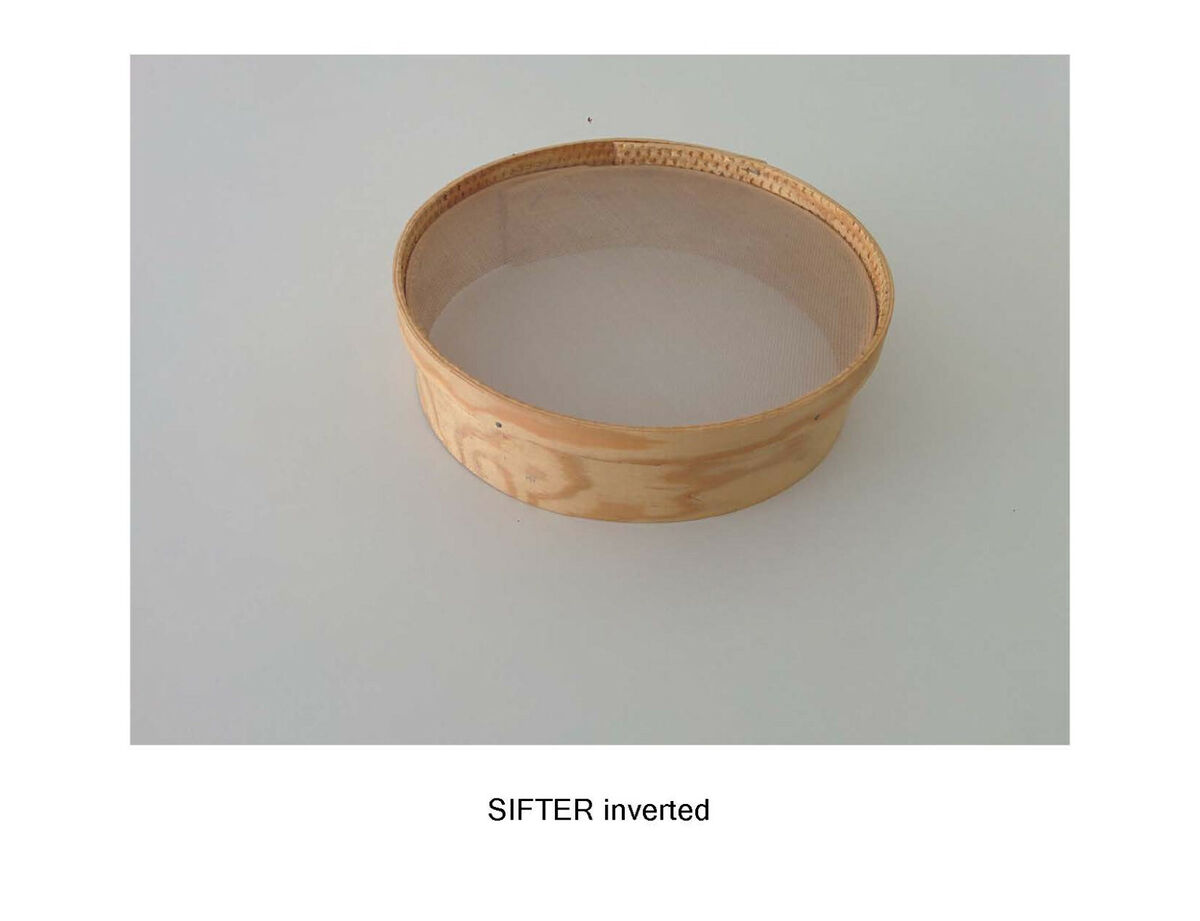This full-color photograph presents a square, monochrome image with a gray background. At the bottom center, there is black text that reads "SIFTER" in capital letters, followed by "inverted" in lowercase letters. The focal point of the image is a light-colored wooden ring, possibly made from veneer, which has been finely crafted and appears hollow inside. The wood grain is visible around its base, giving it a natural texture. The wooden ring has engraved texturing around its lip. The ring sits against a white surface, enhancing its visibility and contrast. The overall image seems to portray an inverted sifter, with its utilitarian purpose left to interpretation.